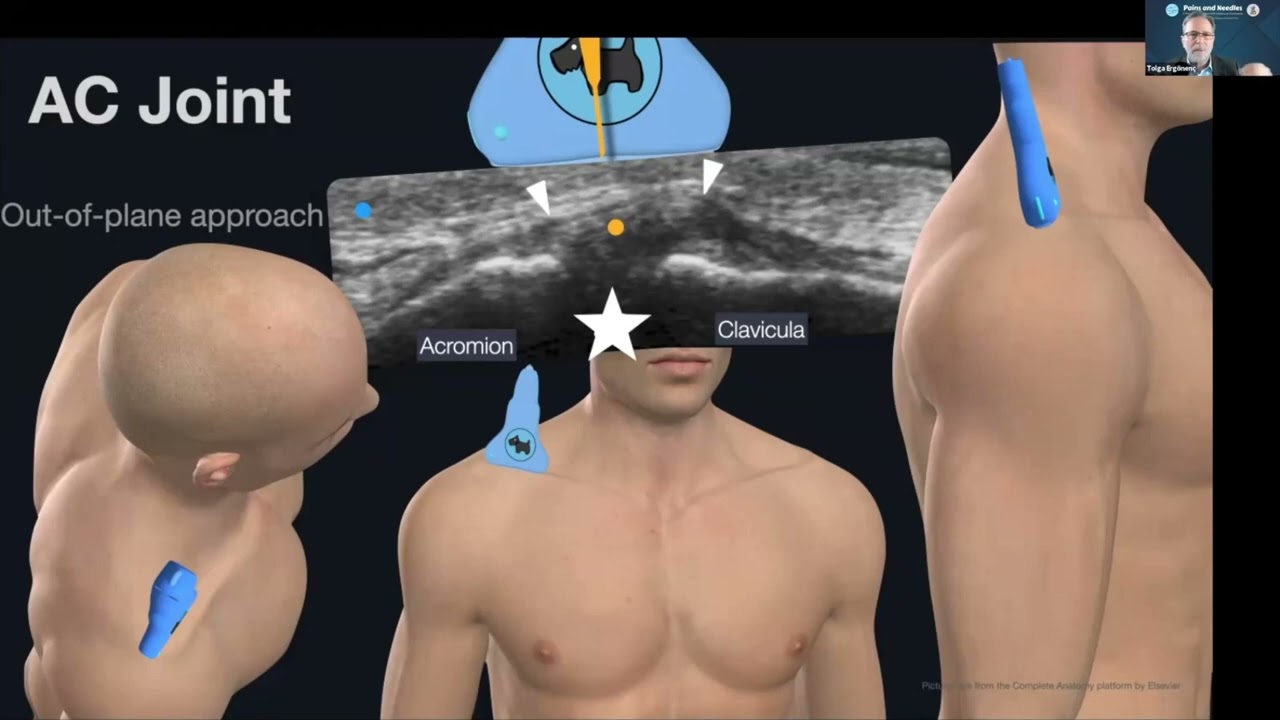The image is a detailed and informative infographic designed to illustrate the anatomy and diagnostic approach to the acromioclavicular (AC) joint using computer-generated human renderings. It features three distinct views of a bald, unclothed male mannequin, each highlighting the right shoulder area where the AC joint is located. The first rendering provides an overhead, transverse view, focusing on the blue-colored AC joint from above the model's head. The second rendering offers a forward-facing view showing the mannequin from the sternum upward, with a clear emphasis on the blue AC joint, though the top of the head is out of the frame. The third image presents a side-profile view of the same blue-highlighted AC joint. The backdrop is black, enhancing the visibility of the models and the blue highlighting. Superimposed over the center view is a black-and-white diagnostic scan, possibly an ultrasound, further pinpointing the AC joint's location. The text "AC Joint Out of Plane Approach" is prominently displayed in the upper left corner of the screen. Additionally, a small thumbnail in the upper right corner suggests a presenter discussing the image, adding an educational context to the visual representation.